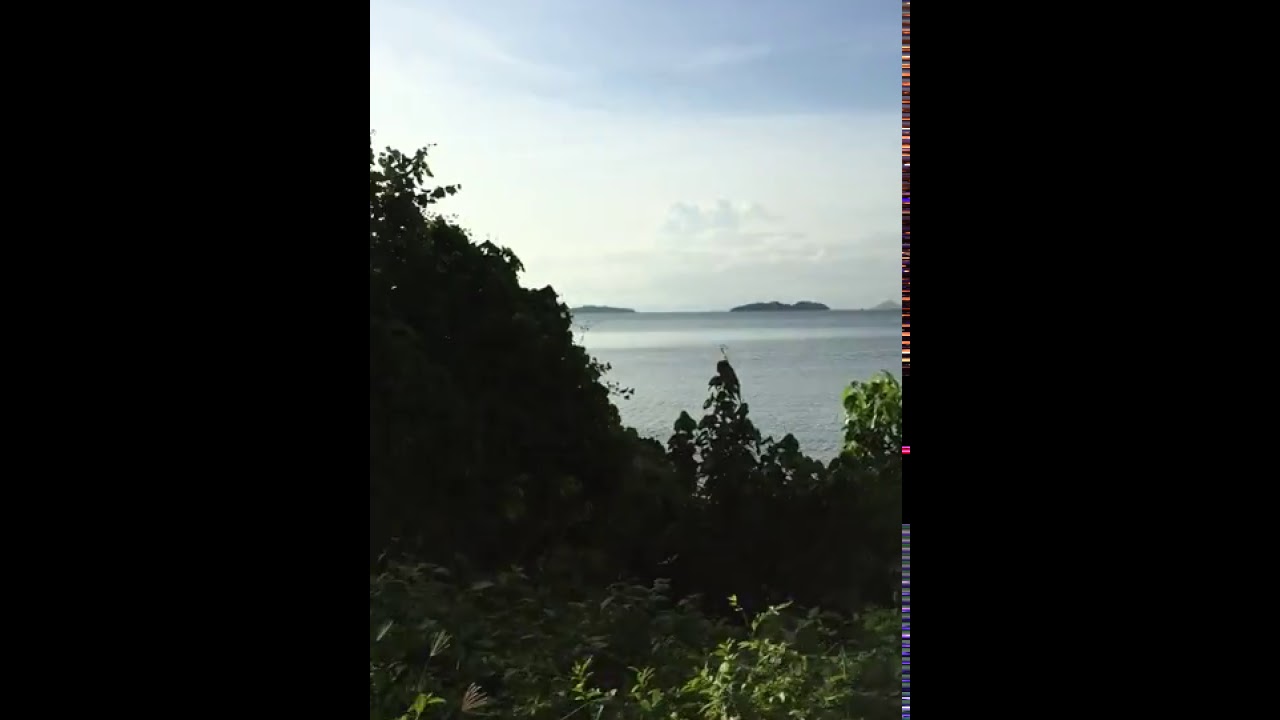The image captures a tranquil island scene overlooking an expansive ocean scape under a daytime sky. In the foreground, dense and lush green foliage, including trees, shrubs, and grass, dominate the view. On the left-hand side, a large plant drapes down towards the center before stretching rightwards across the dense greenery, which is illuminated by faint sunshine peeking through the overcast sky. The middle ground features a vast ocean with gentle waves, exhibiting a light blue tint. Beyond the ocean, three prominent islands or rocky mountainous land masses sit on the horizon. The sky above these islands is mostly gray with some blue patches and large billowing clouds. The image appears to be a vertical one, and there is a notable static-like distortion or discoloration on the right-hand edge, suggesting it may be a scan of a physical photograph.